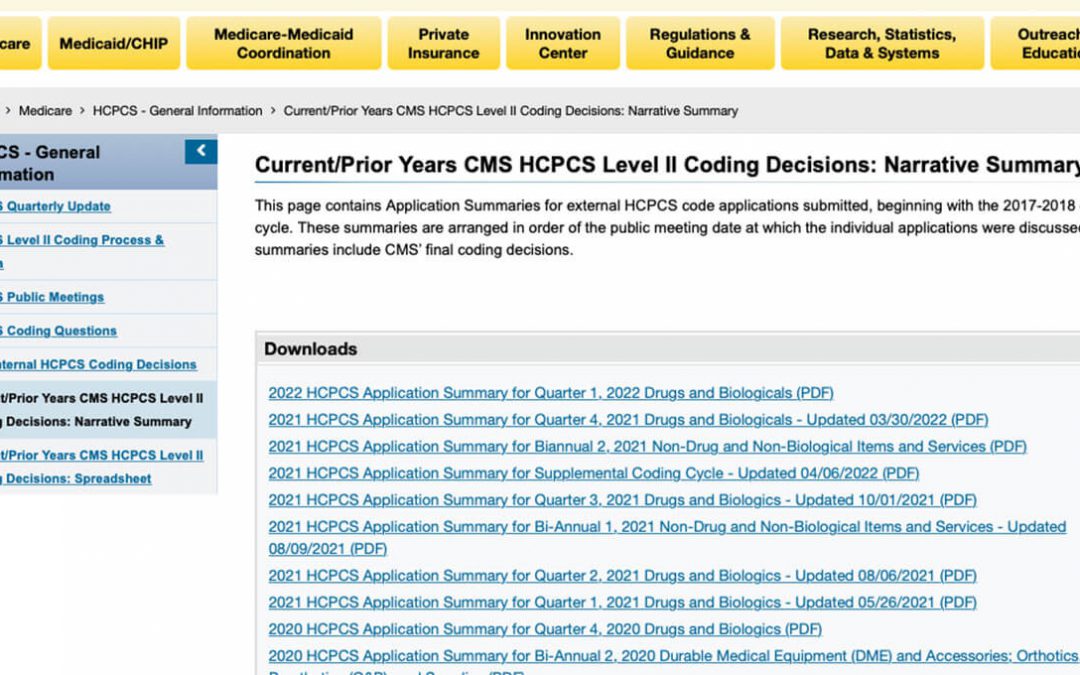Screenshot of a medical website. The top section features several yellow-labeled tabs for different sections including: Medicare/CHIP, Medicare-Medicaid Coordination, Private Insurance, Innovation Center, Regulations & Guidance, Research Statistics, Data & Systems, and Outreach Education.

A menu on the left side displays a dropdown menu, though it's partially cut off and unreadable.

The main body of the page has the heading "Current/Prior Years CMS HCPCS Level II Coding Decisions Narrative Summary." The content below explains that the page contains summaries of external HCPCS code applications submitted from the 2017-2018 cycle onwards. These summaries are organized by the public meeting dates at which the applications were discussed and include CMS's final coding decisions.

There is a box offering downloadable resources with numerous blue hyperlinks. Examples of links include:

- "2022 HCPCS Application Summary for Quarter One, 2022 Drugs and Biologicals (PDF)"
- "2021 HCPCS Application Summary for Supplemental Coding Cycle (Updated 10.01.2021)"